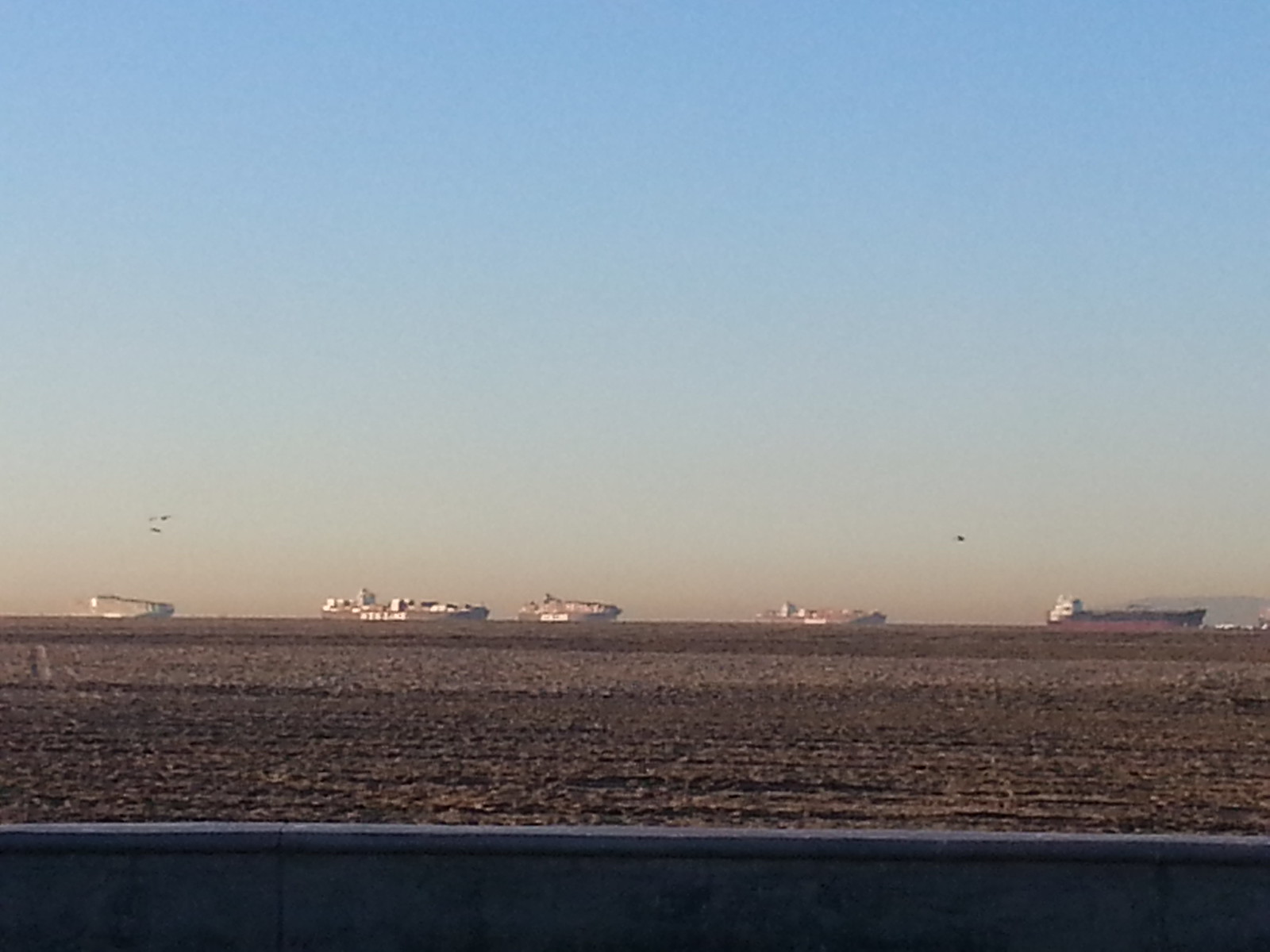The image depicts a coastal scene during sunset, highlighted by a beautiful gradient sky that transitions from blue at the top to a pinkish-orange hue near the horizon. In the midground, a long stretch of meticulously groomed, dark brown sand beach stretches across the frame. Five tanker ships, varying in length and size, are aligned in the distant sea. The foremost ship features a white top where the crew resides and a dark grey front, while the others display shades of grey and white. There is some spacing variation between the ships, with the second and third ships being particularly close together compared to the others. The photo appears to have been taken from a balcony or patio, as indicated by a fence or retaining wall in the immediate foreground. Beyond the ships, a distant hill adds depth to the scene, reinforcing the sense of distance and tranquility.